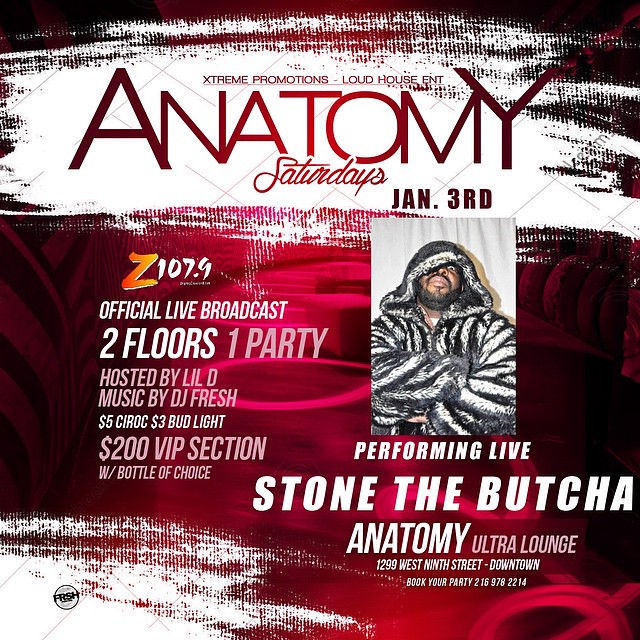The poster, set against a striking red background with elements resembling smeared white paint and little red circular designs, advertises an event at the Anatomy Ultra Lounge, located at 1299 West 9th Street, downtown. Dominating the poster is an eye-catching image of a man clad in a fluffy gray and black fur coat with a hood, beard, and piercing gaze directed at the camera. The promotional text, primarily in bold, reads: "Extreme Promotions" and "Loud House Entertainment" at the top, followed by "Anatomy Saturdays Jan 3rd". Below the central image, the text announces "Performing Live Stone the Butcher" and details the event specifics: "Z 107.9 Official Live Broadcast," "Two Floors, One Party," "Hosted by Lil D," with "Music by DJ Fresh". Additional enticing offers include $5 Ciroc, $3 Bud Light, and a $200 VIP section with a bottle of choice. Contact information for party bookings is also provided: "216-978-2214."